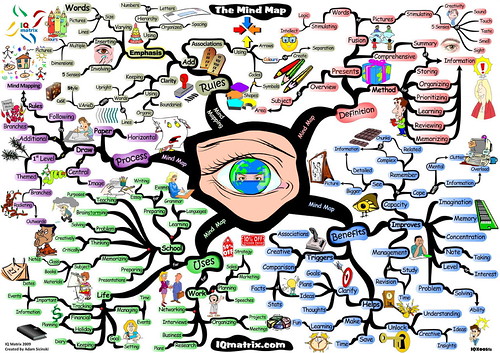The image depicts an intricate "mind map" chart, set against a white background that is largely obscured by a multitude of colorful lines and detailed sections. At the center of the composition is a close-up of an animated eye, with a globe replacing the pupil, featuring green land masses and blue water. Encircling the eye is a thick black outline from which black tendrils extend outward, connecting to various sections of the mind map. These sections, identified by both colors and labels, include "definition" in red, "benefits" in purple, "uses" in green, "processes" in pink, and "rules" in beige. Each section contains further detailed information and small images relevant to the topics, such as a keyboard in the "memory" area. The chart's title, "Mind Map," is prominently displayed in white text on a black squiggly background at the top. The overall image is visually busy, resembling a complex roadmap with elements illustrating different facets of learning and knowledge.